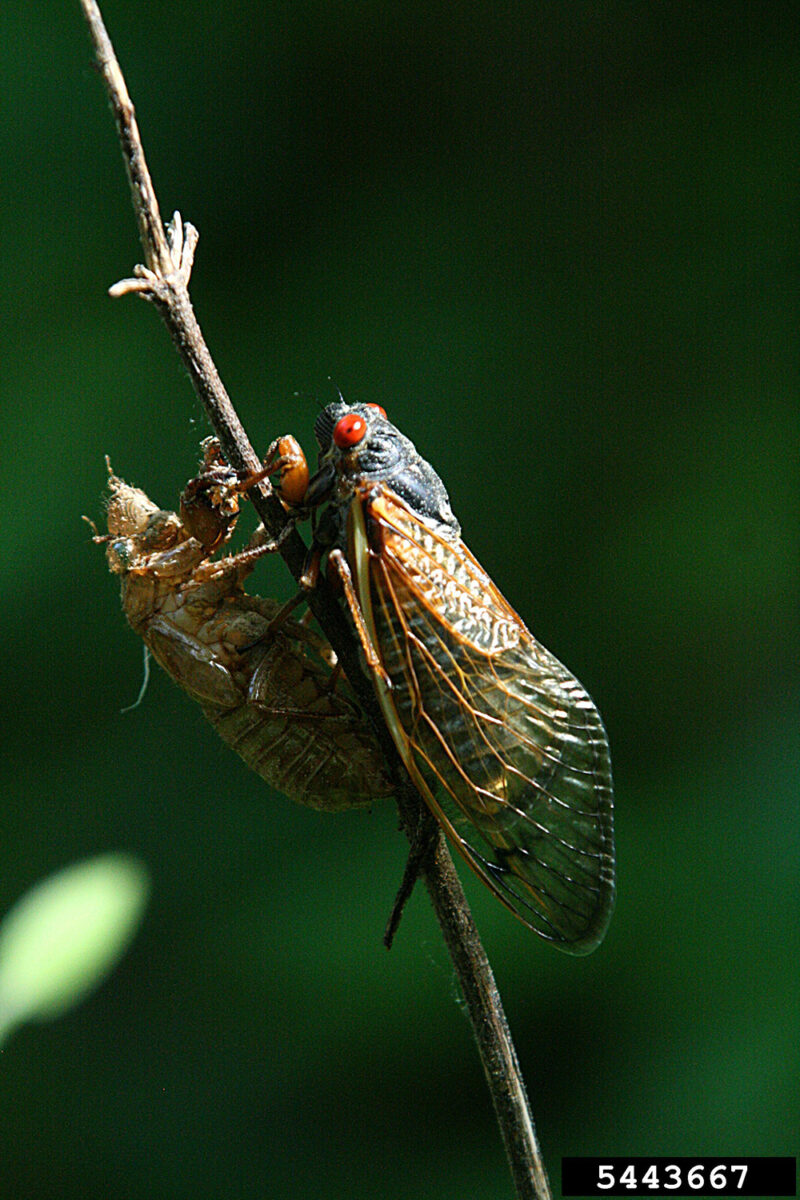This image captures a detailed moment of an insect, likely a cicada or a katydid, perched on a single stick extending diagonally from the bottom center towards the top left of the photograph. The insect exhibits bright red eyes with black centers and has a predominantly black body. Its wings gracefully drape downwards, transitioning from yellow and orange hues to a dark green, with semi-translucent sections accented by visible veins.

The insect is shown from a side view, holding onto the branch with a firm grip. Directly opposite it on the branch is its recently shed, hollow exoskeleton - a light brown or yellowish casing, indicating it has just emerged and is larger than its former shell. Both the insect and its exoskeleton are in sharp focus, contrasting against the blurred, various shades of green background.

At the bottom of the photograph, a black bar with white text displays the numbers 544-3667, adding an additional detail to the captured scene.